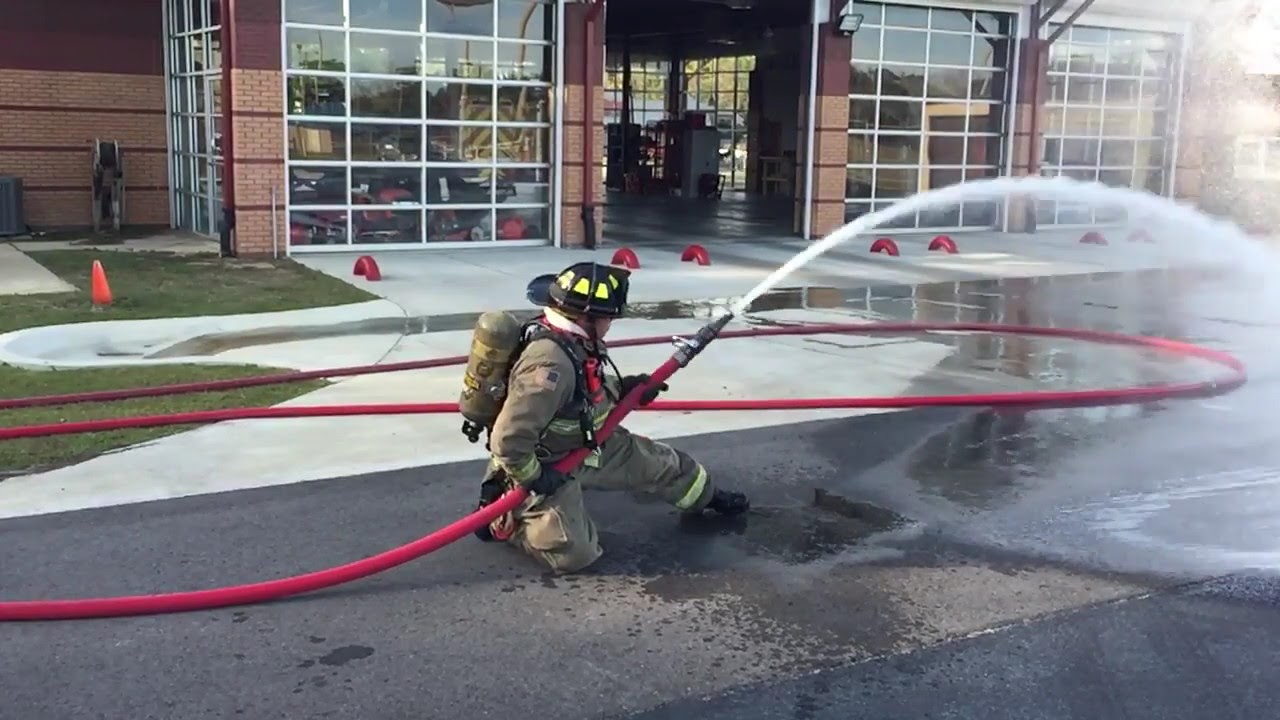In a brightly lit exterior scene, a firefighter is captured in front of a pristine firehouse, featuring one glass door open and three others closed, framed in white. The firefighter, dressed in full gear including a black helmet with yellow markings, khaki or gray suit with reflective yellow-green stripes, heavy boots, and an oxygen tank on his back, is kneeling on the dry pavement. He is holding a red hose, which extends across the scene, and is spraying a powerful stream of water about 20 to 30 feet away. The area around the firehouse is well-maintained, with safety cones positioned in front, and the scene appears to be part of a training exercise on a sunny day. Various fire apparatus, including a fire truck and an emergency truck, can be discerned in the background inside the firehouse.